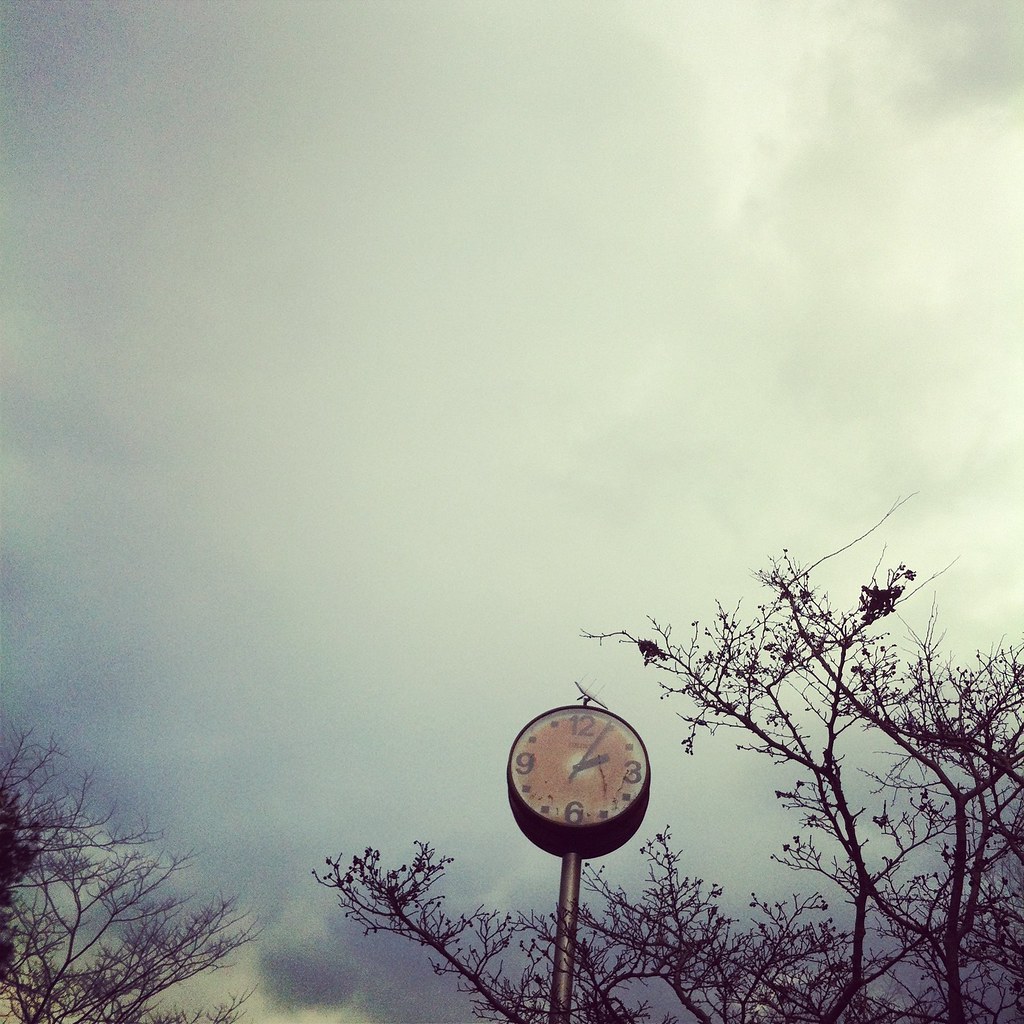This artistic photograph captures a stark, almost melancholic scene. At the center of the image is a round, black clock mounted on a sleek silver pole. The clock's face, heavily dirtied with orange grime, is off-white and features only the cardinal numbers—12, 3, 6, and 9—rendered in black. Black dots mark the other hours, and the clock hands are also black, standing out against the grimy background. The atmosphere is dreary; thick gray clouds blanket the sky, casting a subdued light over the scene. On the left side of the image, tree branches, almost entirely bare, stretch out against a backdrop of dark gray clouds. Similarly, on the right side, more barren trees, with scant leaves, add to the somber mood. The photo quality is excellent, displaying an artistically grainy texture that enhances its haunting beauty.